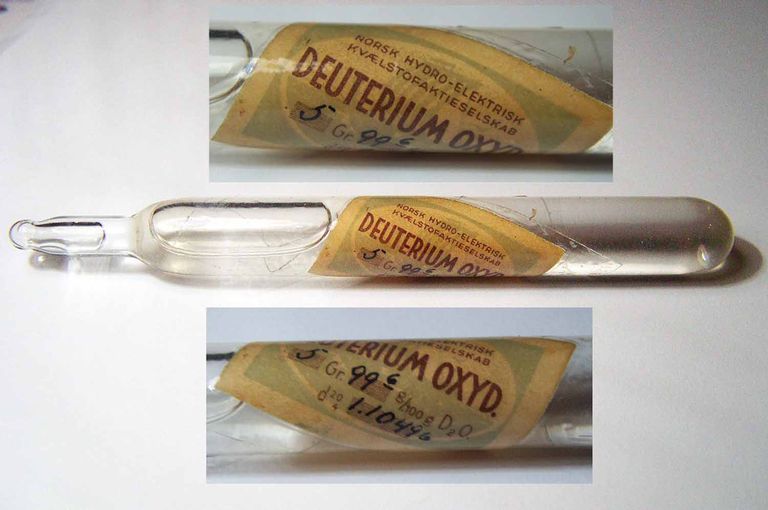This is a color photograph in landscape orientation depicting a glass vial filled with a clear liquid, displayed horizontally against a light gradient gray background that is lighter on the left and darker on the right. The vial, centered both vertically and horizontally, features a narrow pointed end on the left and a rounded bottom on the right, positioned perfectly horizontal. Prominently wrapped around the center of the clear, smooth glass cylinder is a faded, pale yellow label with bold, capital red text reading "DEUTERIUM OXYD." This label is diagonally oriented around the vial and also includes difficult-to-read smaller red text in a foreign language, possibly "Norsk Hydroelektrisk," among other details. Handwritten in black marker, the label displays the numeral "5" followed by measurements and data, including "TR 99.6" and "1.1044." Enhancing the visibility of the label's details, there are two photographic inserts positioned above and below the vial, offering close-up views of the upper and lower portions of the label, reflecting a style of photographic representational realism.